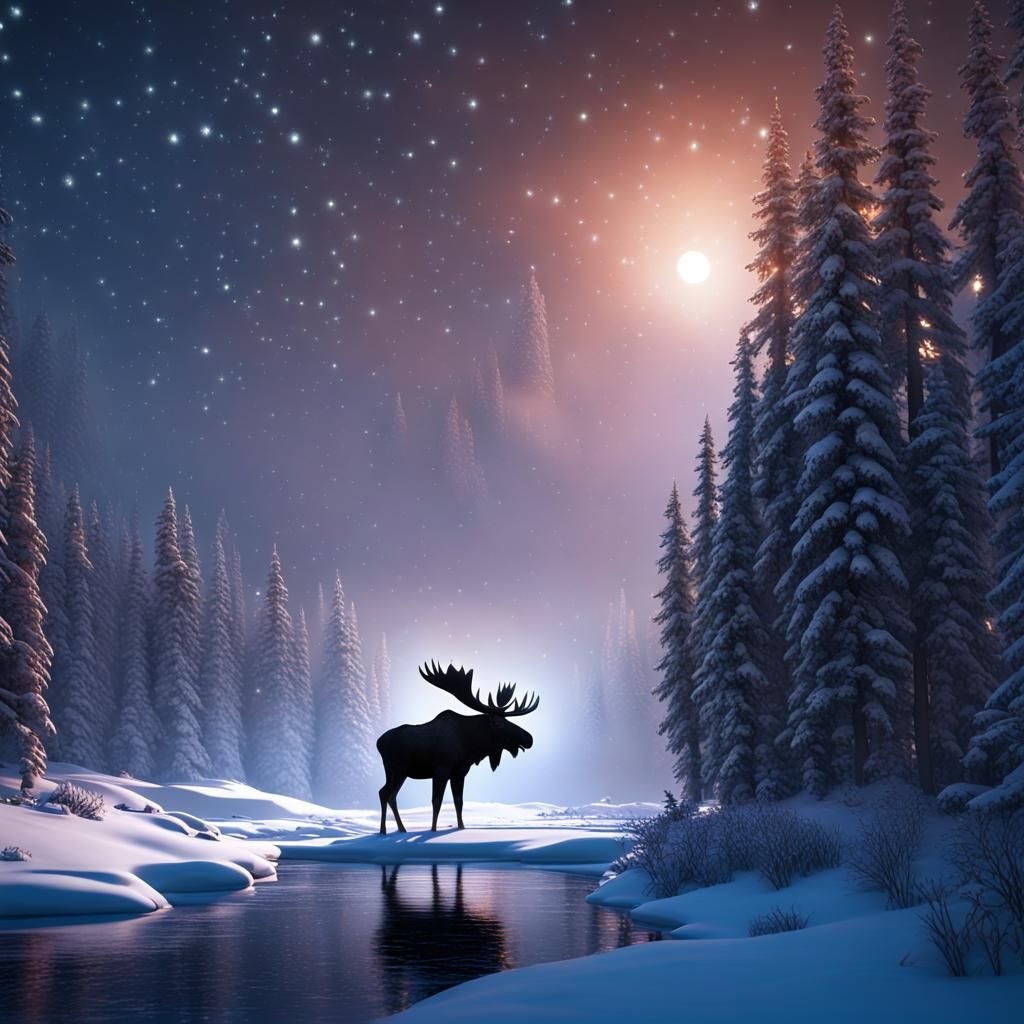In a digitally created, mystical nature scene, the silhouette of a bull moose with large, dramatic antlers stands prominently in the lower center against a pristine, snow-covered landscape. Its strong body and long legs are striking against the untouched snow, which shows no footprints. The moose is positioned just before a glass-like, flat water body, possibly a small, frozen lake. Surrounding the moose are tall, evergreen trees with branches heavily laden with snow, adding to the serene and calm atmosphere. The sky above is a jet-black canvas sprinkled with twinkling stars and illuminated by a bright, nearly sun-like moon. Adding to the surreal and calming ambiance, there is a mist effect that envelops the scene, making it even more enchanting. Interestingly, in the sky, some coniferous trees appear to float, adding an otherworldly touch. The moonlight casts an ethereal glow behind the moose, subtly revealing the outlines of distant peaks, making the entire artwork feel like a peaceful yet otherworldly wilderness.